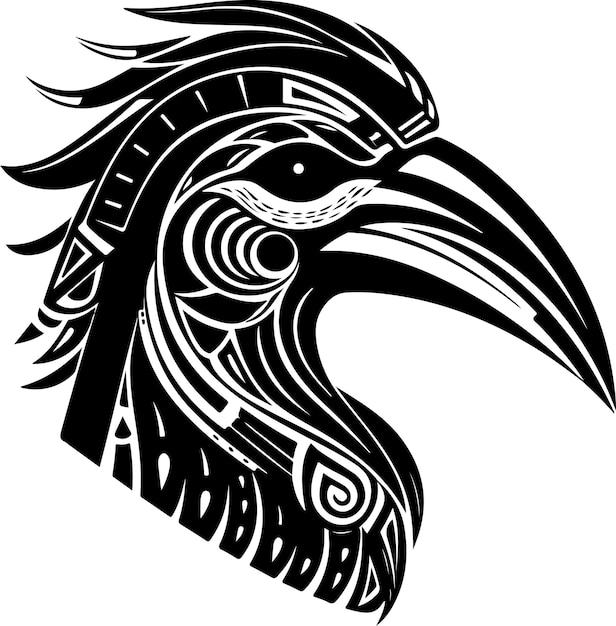This black-and-white image features a detailed, stylized sketch of a bird's head in profile, seemingly combining elements of impressionist and Native American art styles. The bird is facing to the right, showcasing one prominent eye with a white dot set in an entirely black eye. The head is adorned with intricate feather details, particularly on top and along the neck area, which is decorated with geometric designs. The beak is long, sharp, and curved, adding to the impression of the bird being a bird of prey. Notably, the feathers extending from the back of its head resemble a mohawk or crest, giving the bird a striking appearance. The background is completely white, and the bird itself is rendered in bold, blocky sections of black ink, resembling a print from a computer printer. No watermarks, artist signatures, or any other writings are present, emphasizing the simplicity and focus of the artwork.